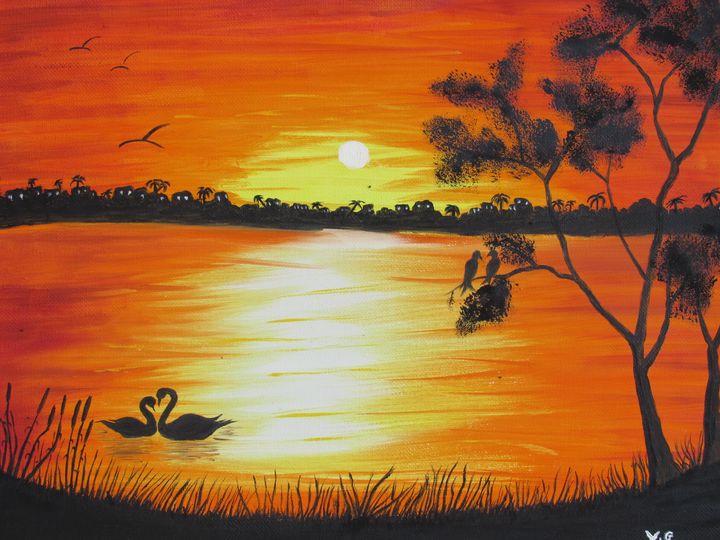In this elegant and realistic painting, the vivid sunset dominates the scene with an orange and yellow sky, casting a warm glow over everything. The sun, setting near a large pond or perhaps a giant lake, bathes the water in hues of orange and yellow, creating vibrant reflections. Surrounding the water, dense trees and tropical palms frame the composition, some appearing as dark silhouettes against the bright sky. Birds, including several geese or swans, are seen gliding across the water or flying above, their forms rendered in black due to the backlighting of the setting sun. In the distance, small houses with tiny lit windows are nestled amongst the trees, adding a hint of life to the serene landscape. The scene is pulling towards dusk as the darker tones take over the bright sky, indicating the imminent approach of nighttime. This richly detailed image captures a tranquil and enchanting moment in time, further accentuated by subtle details like the signature VG in the bottom right corner.